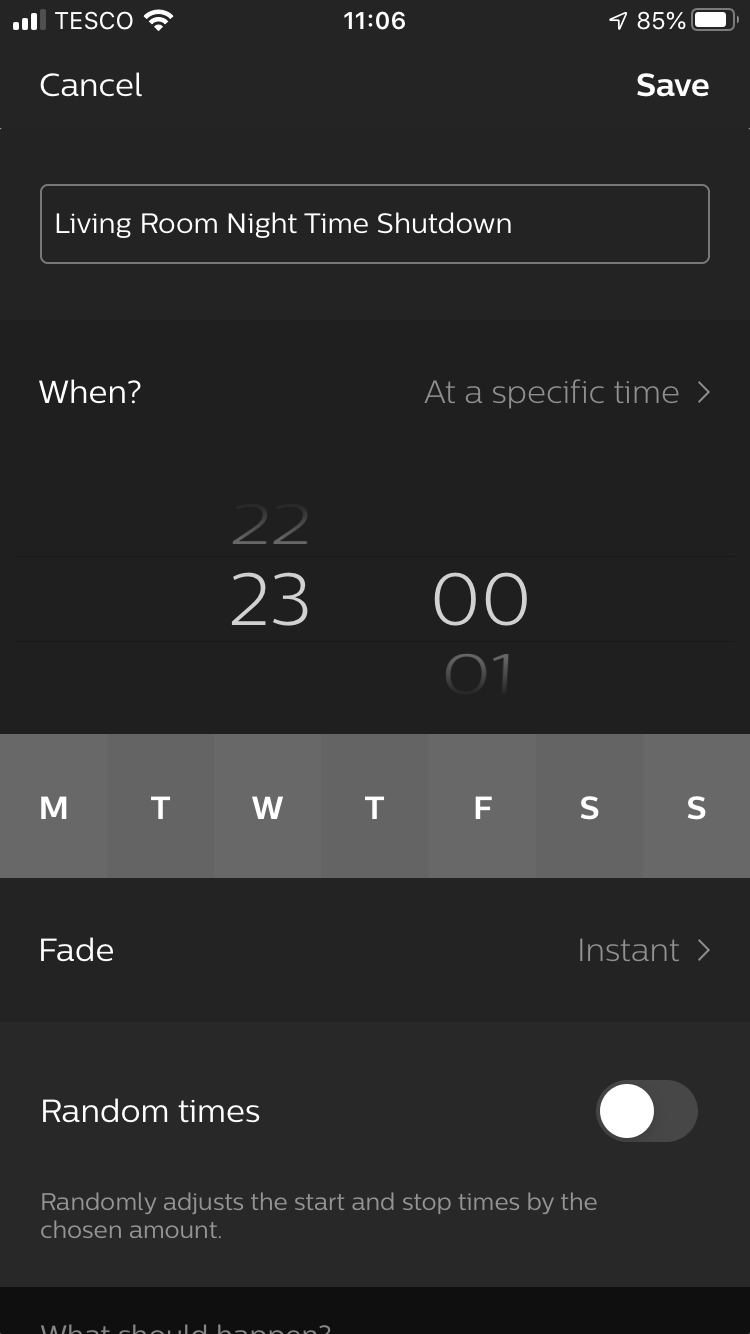Screenshot Description:
The screenshot features a smartphone interface with a black background. On the upper left-hand side, the word "Tesco" is displayed in white, accompanied by two Wi-Fi symbols. Centrally, the time "11:06" is prominently shown. On the upper right, there is an icon depicting an arrow pointing to the right, next to the battery status indicating 85% remaining. Below "Tesco," there are options labeled "Cancel" and "Save" written in white.

Beneath this section is a gray-outlined text box with a white font that reads "Living room night time shutdown." Beneath this text, it says "When?" in white, and to its right, in a lighter gray, there are the words "At a specific time" followed by a right-pointing arrow.

Following this segment is a scrolling numerical interface, currently set to the number "23" on the left, with "00" to the right of it, precisely centered. The numbers "22" and "01" are partially visible above and below their respective counterparts, suggesting a scrollable wheel function.

Below the numerical interface are the abbreviations for the days of the week: "Mon," "Tue," "Wed," "Thu," "Fri," "Sat," and "Sun," each in block format with alternating shades of gray and white font.

Further down, the option "Fade" is presented on the left, while "Instant" is displayed on the right accompanied by a right-pointing arrow. Beneath this, there is a toggle button next to the label "Random times," which is currently switched on. At the bottom of the screen, a description in light gray states, "Randomly adjust the start and stop times by the chosen amount," providing additional context for the random times feature.